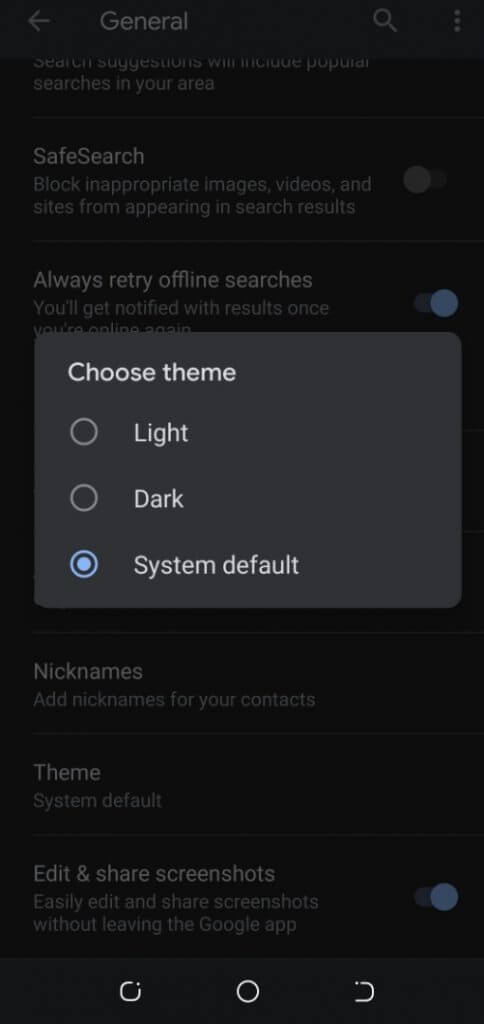A cell phone screen displays an app in dark mode, making the background black. Gray text contrasts against the dark setting. A semi-transparent overlay darkens the screen further, ensuring focus on a prominent floating dialog box in the center. 

The dialog box, in a charcoal gray hue, is titled "Choose Theme." It features radio buttons for theme options: light, dark, and system default. The user has selected the "system default" option. The dialog also shows several settings: 

- Safe Search is turned off.
- "Always retry offline searches" is enabled.
- There are no nicknames listed.
- The Theme setting is confirmed as "system default."
- The option to "Edit and share screenshots" is turned on.

At the bottom of the screen are navigation buttons, which appear distinct. The center button features a circle with a break and a backward "C" shape, whose functions are unclear.